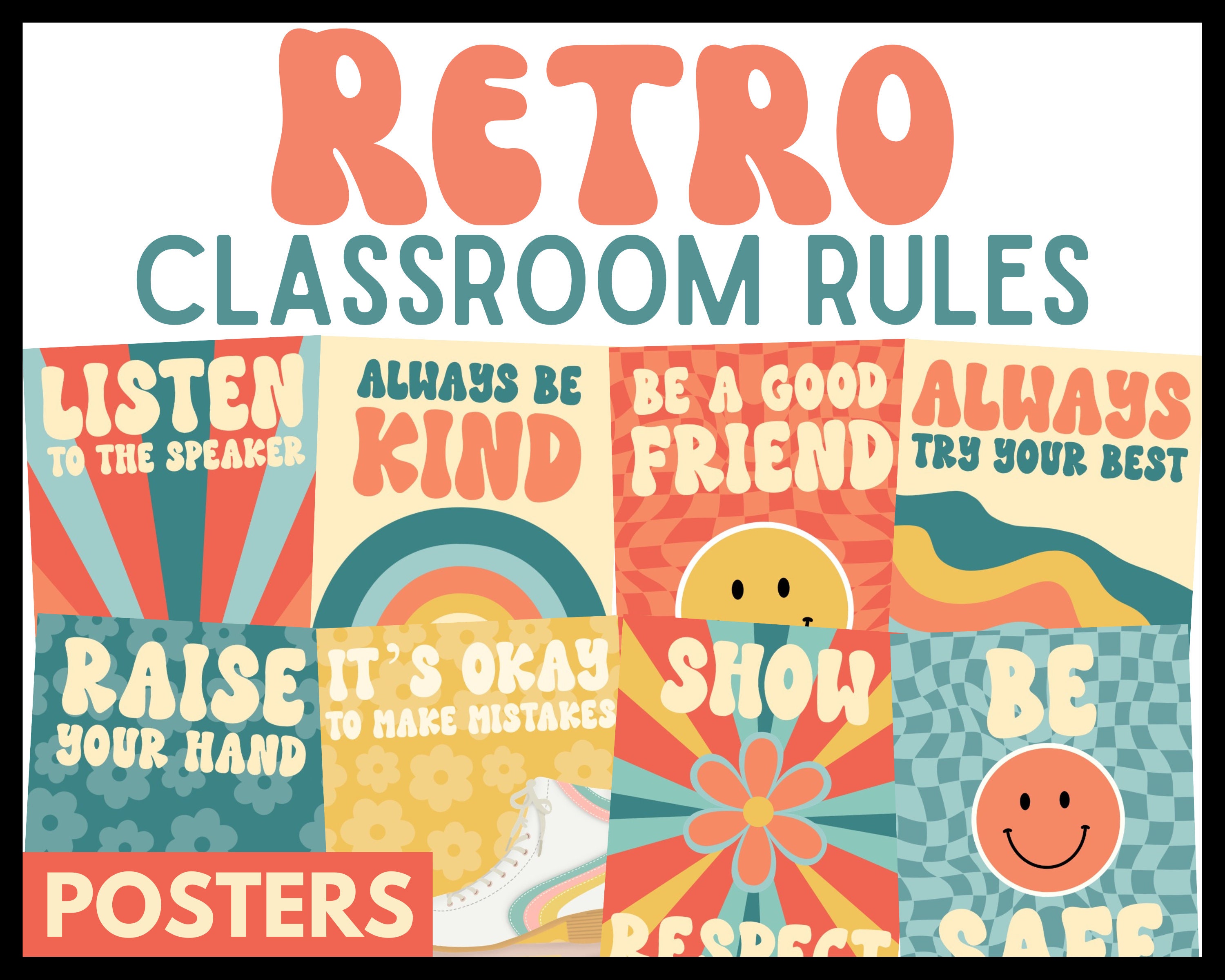This poster is titled "Retro Classroom Rules" with "Retro" prominently displayed in a bold, 70s style orange font, and "Classroom Rules" in a contrasting green color. Below the title, eight creatively illustrated cards list the following rules: listen to the speaker, always be kind, be a good friend, always try your best, raise your hand, it's okay to make mistakes, show respect, and be safe. Each card is decorated in muted colors like aqua, peach, yellow, orange, and pink, featuring vintage-style illustrations such as retro shoes, smiley faces, and rainbows, further enhancing the nostalgic 1970s vibe. In the lower left corner of the poster, the word "posters" confirms that this is indeed a poster.